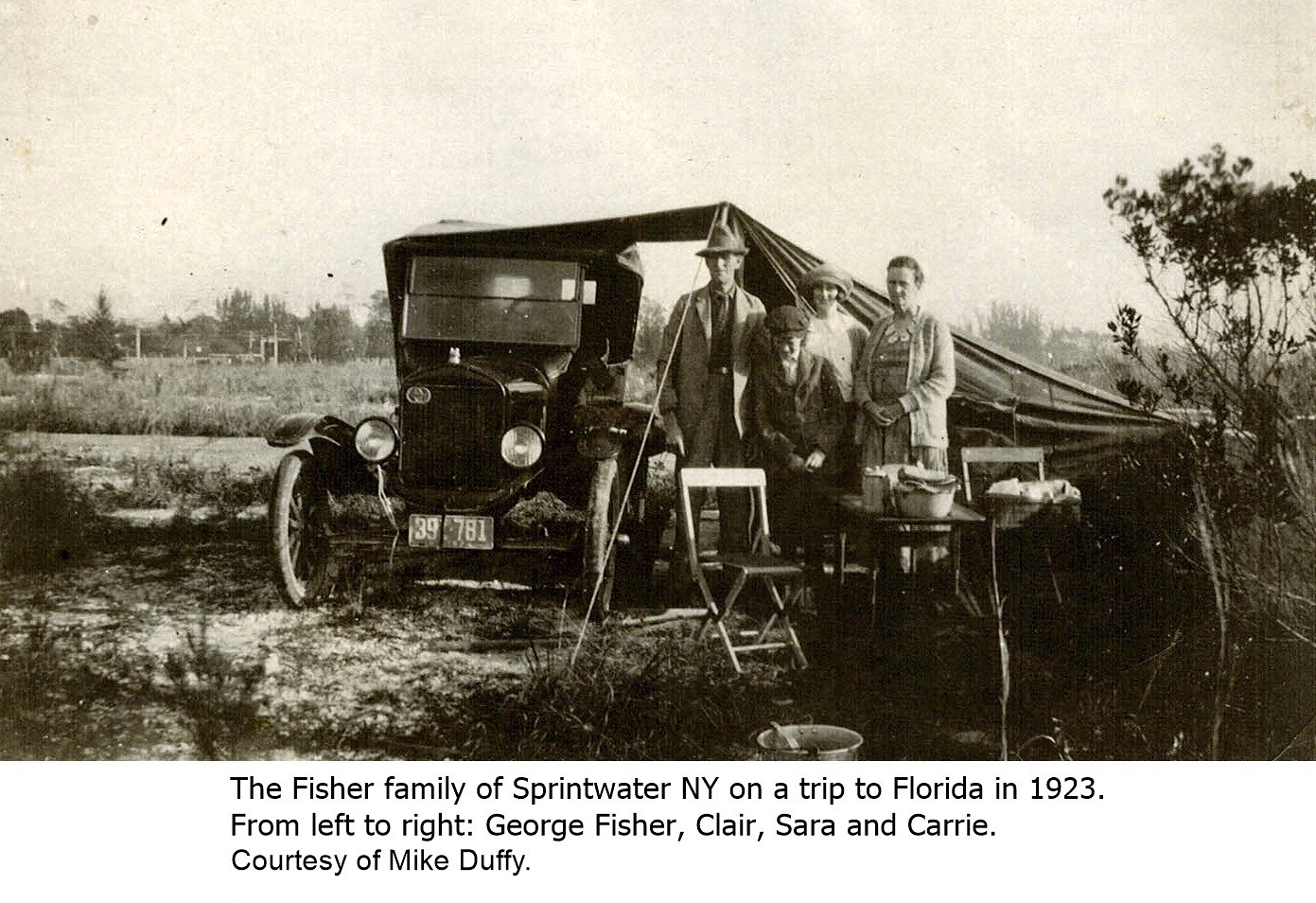This vintage black and white photograph, with a heavy sepia tone, captures the Fisher family from Sprintwater, New York, during their trip to Florida in 1923. The caption beneath the image reads: "The Fisher family of Sprintwater, New York, on a trip to Florida in 1923. From left to right, George Fisher, Claire, Sarah, and Carrie. Courtesy of Mike Duffy."

The image shows the family posing in an outdoor setting. On the far left stands George Fisher, a tall man wearing a fedora hat, a light-colored jacket, and a dark shirt. Next to him is Claire, a young child donning a hat and jacket, possibly a boy. Behind Claire, slightly towards the center, stands Sarah, a middle-aged woman with fair skin, her hair pulled back, dressed in a printed dress paired with a cardigan-style jacket. On the far right is Carrie, the eldest woman, wearing a dress and standing slightly apart from the group.

In the foreground, there is a simple table, possibly a folding card table, cluttered with pots, plates, and other items, suggesting a picnic or outdoor meal. Two empty folding chairs are positioned around the table. To the left of George is an old black automobile with high wheels and large, rounded headlights, angled slightly towards the camera. Behind the family and extending to the right edge of the photograph is a makeshift tent, whose exact support structures are unclear.

The setting appears to be a grassy field with patches of dirt and weeds, and in the background, a dense line of trees defines the horizon under a clear, sunny sky. The overall scene reflects a moment of calm and simplicity from the early 20th century, preserved in this timeless photograph courtesy of Mike Duffy.